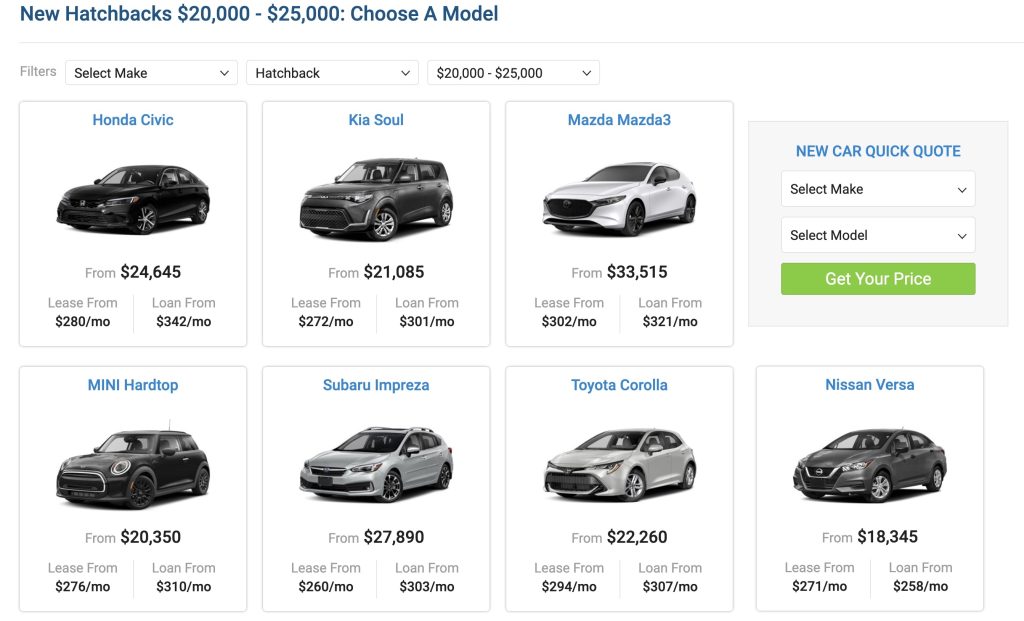This image is a comprehensive advertisement for new hatchbacks, showcasing seven different models available within the price range of $20,000 to $25,000. 

In the top left corner, written in dark blue text, the heading reads: "New Hatchbacks $20,000 to $25,000, Choose a Model." Below this, a user interface allows filtering by make, vehicle type (hatchback), and price range.

Displayed are the images and details of seven hatchback models:
1. **Honda Civic** - Black, priced from $24,745. Lease options start at $280 per month, and loan options at $242 per month.
2. **Kia Soul** - Black, priced from $21,085. Lease options start at $272 per month, and loan options at $211 per month.
3. **Mazda 3** - White, priced from $32,415. Lease options start at $222 per month, and loan options at $221 per month.
4. **Mini Cooper Hardtop** - From $30,350. Lease options start at $276 per month, and loan options at $210 per month.
5. **Subaru Impreza** - Silver grey, priced from $27,890. Lease options start at $260 per month, and loan options at $233 per month.
6. **Toyota Corolla** - From $22,260. Lease options start at $294 per month, and loan options at $307 per month.
7. **Nissan Versa** - Dark grey, priced from $18,245. Lease options start at $271 per month, and loan options at $238 per month.

The names of the cars are written in blue, while the prices are in black. Positioned at the top right is another section titled "New Car Quick Quote." It invites users to select a make and model to get the price, with the "Get Your Price" button highlighted in green. The background of the image is white, ensuring the relevant information is easily legible.